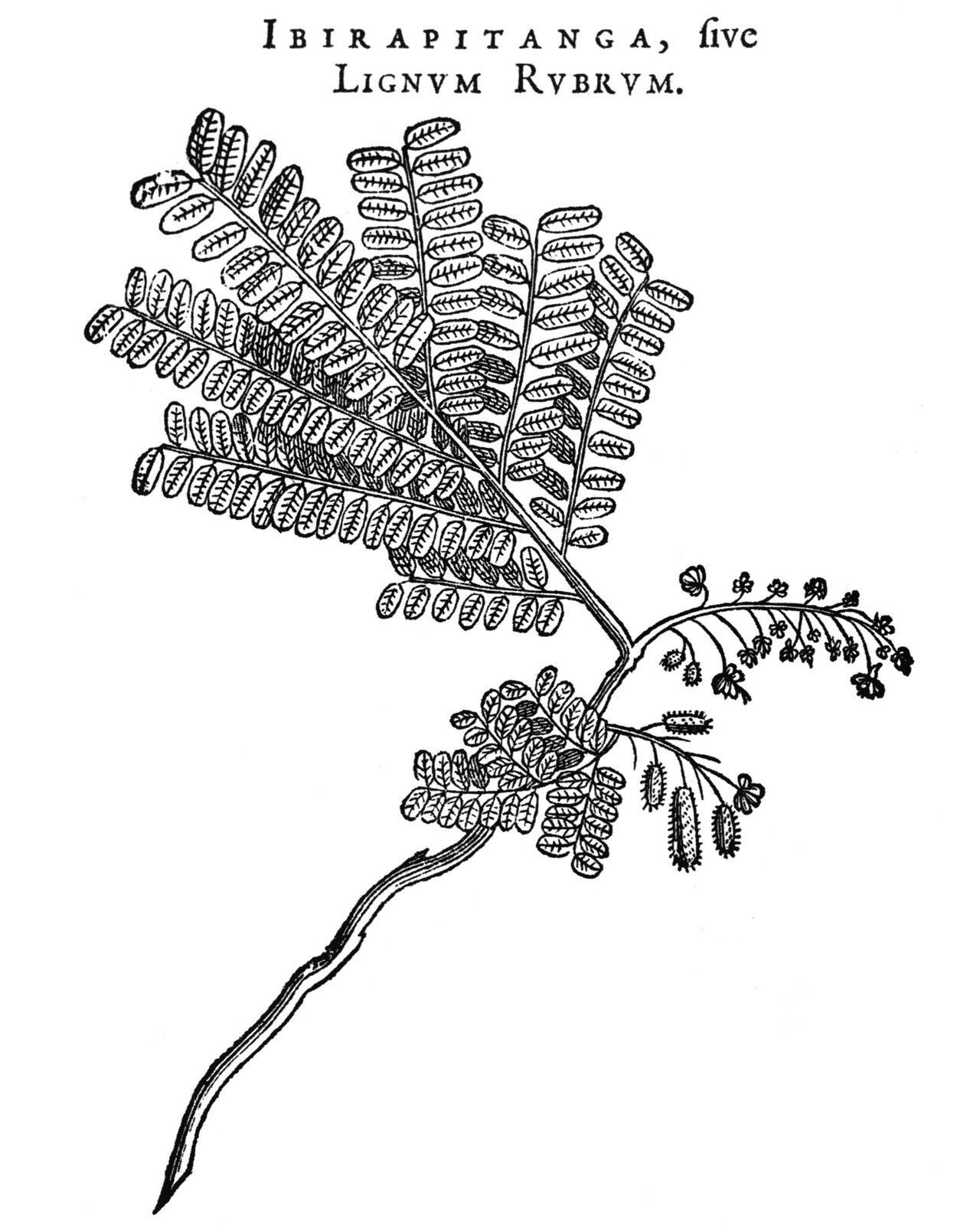The hand-drawn black-and-white illustration depicts a branch emerging from the lower left corner of the image and extending upwards to the right, eventually splitting into three distinct smaller branches. The largest of these smaller branches extends back towards the upper left corner, while the other two extend horizontally towards the right. Each branch is adorned with numerous small leaves and tiny flowers clustered along their lengths. The background of the illustration is entirely white. Intricately detailed, the drawing includes some spiky seed pods along with the delicate leaves. At the top of the image, there is an inscription in black ink that reads "Ibera pitanga, 5 Lignum rubrum," which appears to be a scientific or botanical name, enhancing the impression that this is a botanical illustration one might find in a reference book.